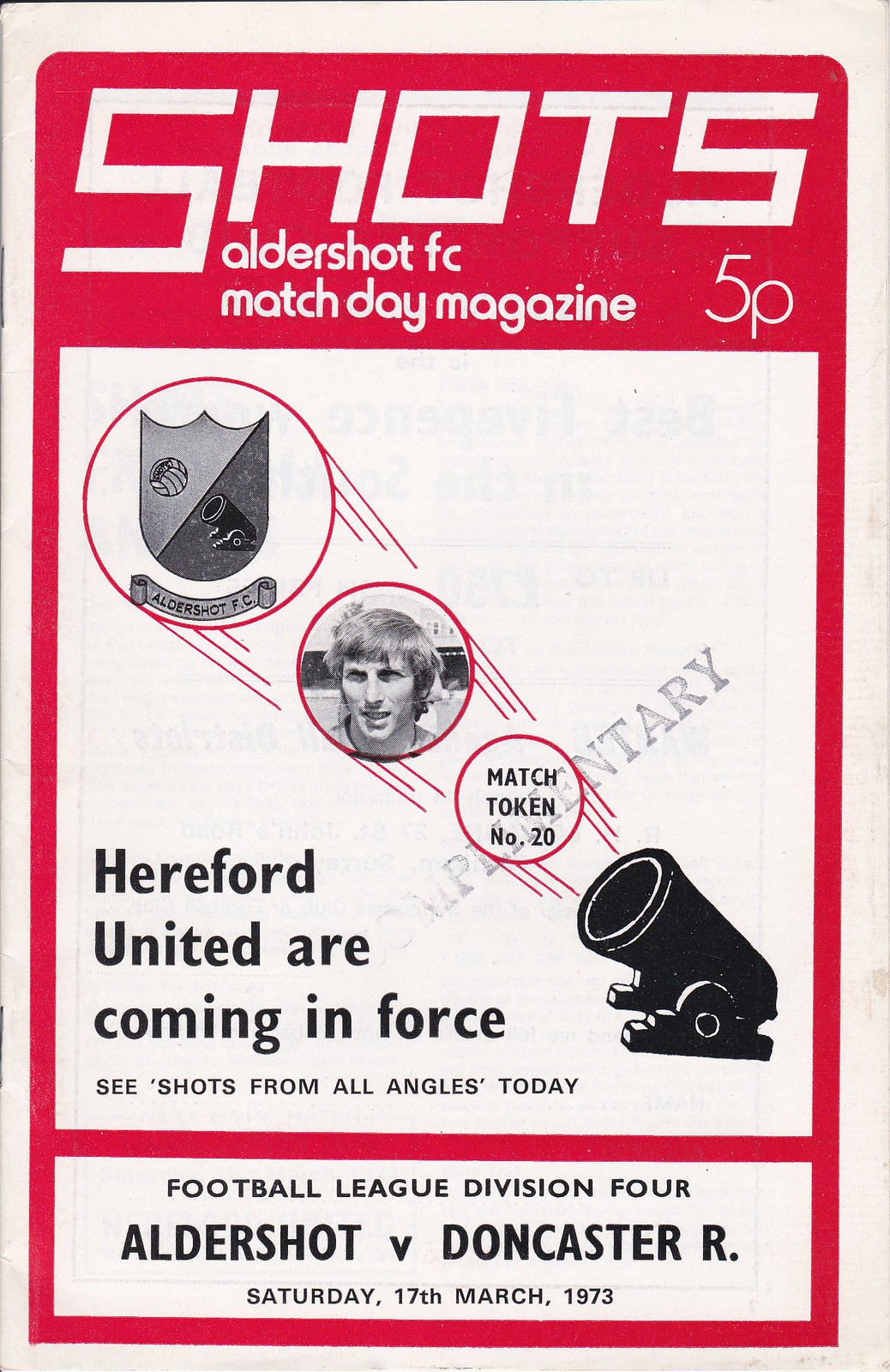The image showcases a vintage cover of a soccer program, specifically the match day magazine for Aldershot Football Club titled "Shots." The magazine, dating back to March 17, 1973, has a distinctive design with a red border outlining all text and images. At the top of the cover, written in bold, white italic letters on a heavy red horizontal bar, is the word "Shots." Just beneath, in smaller lowercase white text, are the words "Aldershot F.C.” followed by "Match Day Magazine." The price is listed as “5p.”

Central to the cover is a stylized black cannon pointing upwards to the left, with three red-outlined circles emerging from its mouth, symbolizing shots. The circles vary in size, diminishing as they move upwards. The largest circle, located in the upper section, contains a gray shield with a diagonal divide, featuring crests on both halves and a banner underneath, although the text is too small to read. The middle circle houses a black-and-white photograph of a clean-shaven young man with longish blonde hair, likely a player, standing in front of a stadium. The smallest, lower circle contains the black text "MATCH TOKEN NUMBER 20."

Below these circles, on the left side, in black text, are the lines “Hereford United are coming in force” and “See shots from all angles today.” A red horizontal divider follows, with black text underneath that reads “Football League Division Four,” followed by “Aldershot versus Doncaster R” in larger, bolder print. The date “Saturday, 17th March, 1973” is displayed at the bottom. The overall wear and tear on the cover indicate its age, approximately 50 years old.